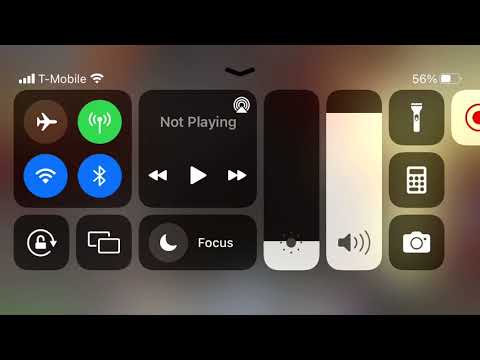This image is a detailed screenshot of an iPhone's control center in landscape orientation with a silver or brushed metallic gray frame. The phone is situated against a black background, accentuated by a black border at the top and bottom of the image. In the upper left corner of the screen, the status bar shows four white connectivity bars, the carrier name "T-Mobile," a Wi-Fi symbol, and a battery icon at 56%. Below the status bar, three distinct sections are observed, predominantly with icons set against black squares or rectangles with rounded corners.

The left section consists of a black square with four circular icons: an airplane, a green icon possibly depicting a microphone, and two blue icons with a white Wi-Fi symbol and an unidentified white blob, respectively. 

To the right of this, a black square displays the media controls featuring the text "Not Playing" in white at the top, above a play button flanked by rewind and fast-forward icons.

Below these squares are three smaller black squares: 
1. A lock icon.
2. Two overlapping squares icon.
3. A crescent moon icon labeled "Focus."

Adjacent to these elements, towards the right, are two vertical rectangles: 
- The left rectangle is black with a small white bottom edge.
- The right rectangle is primarily white with a slight black top edge, depicting a volume bar nearly at its maximum.

Lastly, aligned vertically to the right are four black buttons with icons:
1. (Partially visible) a red circle resembling a bullseye.
2. A flashlight.
3. A calculator.
4. A camera icon.

The overall composition aptly mirrors the interface layout seen when accessing the control center on an iPhone.